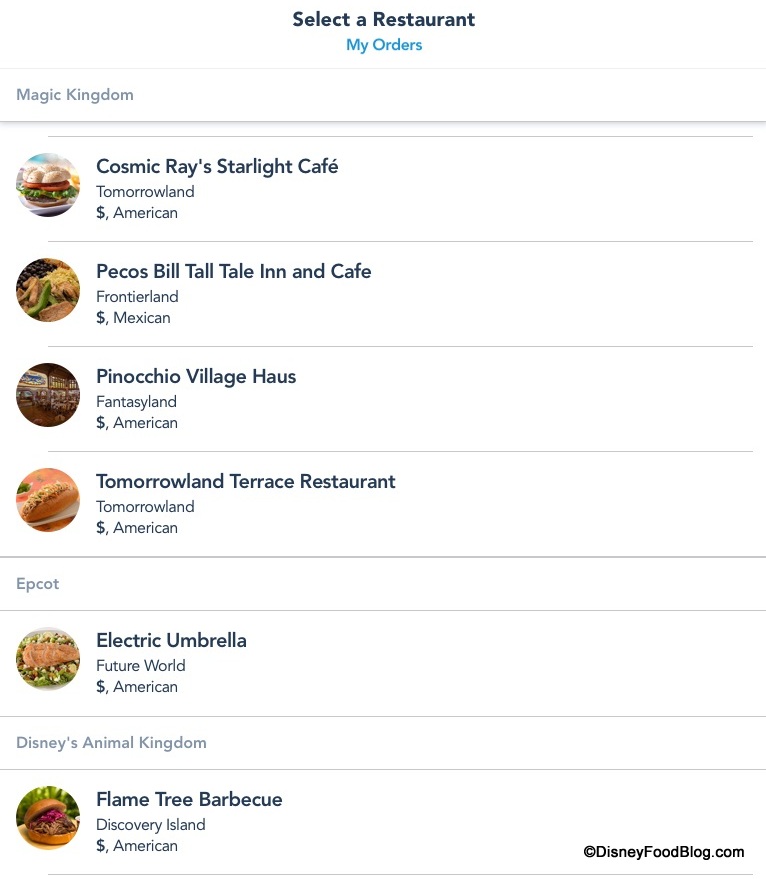Screenshot of a Disney World restaurant ordering interface. Listed locations include Magic Kingdom, Epcot, and Disney's Animal Kingdom. Under Magic Kingdom, four restaurants are selected: Cosmic Ray's Starlight Cafe, Pecos Bill Tall Tale Inn & Cafe, Pinocchio Village Haus, and Tomorrowland Terrace Restaurant. For Epcot, the listed restaurant is Electric Umbrella. For Disney's Animal Kingdom, the featured restaurant is Flame Tree Barbecue. It appears to show restaurants available on a meal plan or similar service. A copyright notice at the bottom reads "DisneyFoodBlog.com."